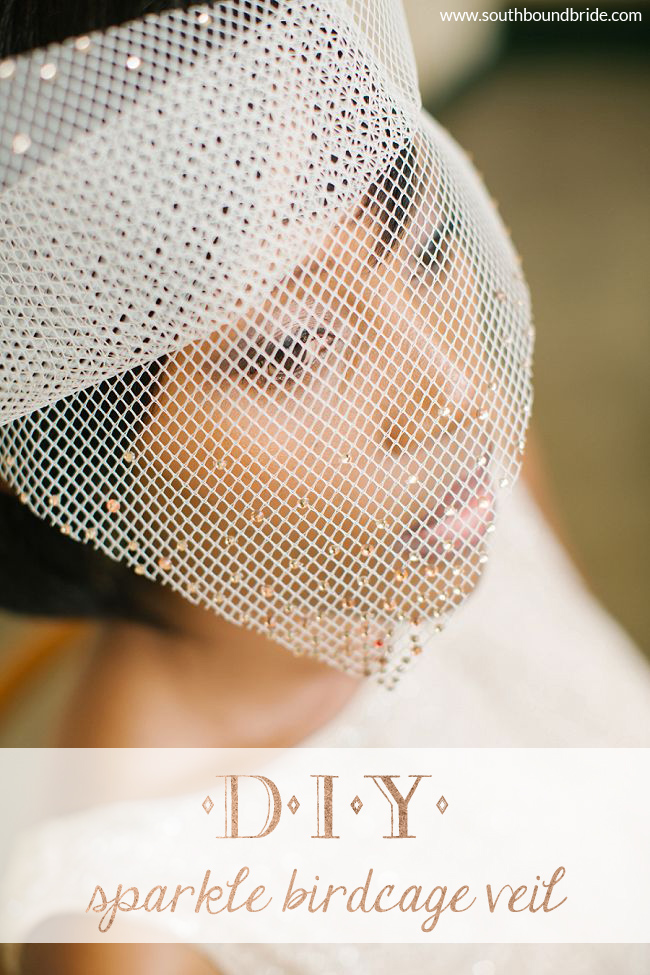The photograph is a professionally shot, full-color image featuring an attractive African-American woman gazing upwards from the left to the upper right-hand corner of the frame. The image is vertically rectangular with a predominantly brown-green, furry background. The woman's visage and a portion of her neck and shoulders are the main focus of the image. She has short dark hair, dark eyes, light pink lipstick, and is wearing a white dress, possibly a wedding gown.

A distinctive feature of the photograph is the intricate sparkle birdcage veil that elegantly covers her face. The veil is a heavy net adorned with tiny, golden-looking faux gemstones that catch the light. It is folded thicker at the forehead, giving it a layered appearance while leaving her chin exposed.

Toward the bottom of the image, there is a prominent white band with text written in brown. It reads, "DIY Sparkle Birdcage Veil" in a mix of bold and cursive fonts. Additionally, the upper right-hand corner of the photo includes a watermark with the URL: www.doubt.southboundbride.com, suggesting that this image is an advertisement or a promotional piece for a do-it-yourself wedding veil product.